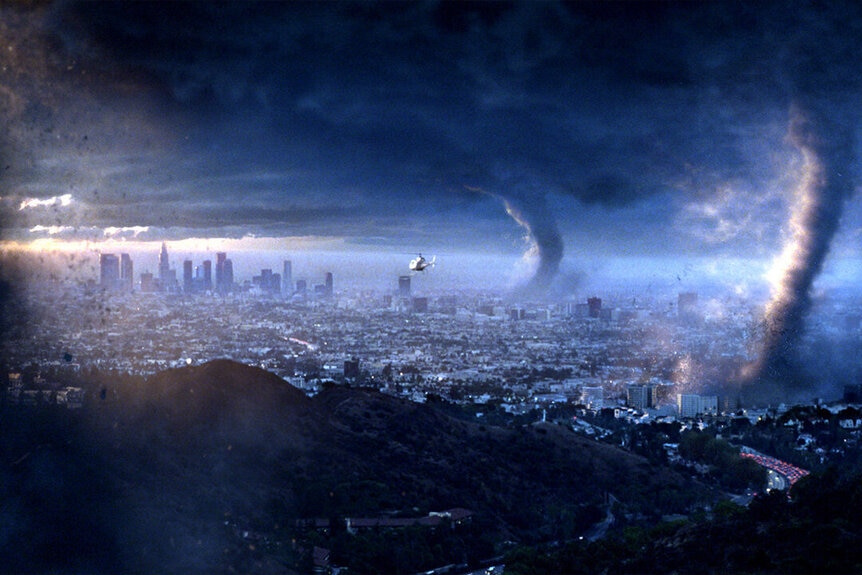The image, almost resembling a painting, depicts a dramatic aerial view of a city like New York or Los Angeles engulfed in a severe storm. Dominating the scene are two tornadoes touching down, one straight and the other slightly bent, creating a sense of movement and chaos. The right side of the image prominently features these swirling tornadoes, surrounded by mist and fuzziness, creating an ethereal atmosphere. In the center, a helicopter flees the unfolding disaster amidst the towering skyscrapers. The skyline is painted with dark, blue and black clouds, intensifying the ominous mood. Light pierces through the left side of the image, providing a stark contrast to the otherwise dark foreground. In the front of the image, there's a small mountain, adding depth. This composite view masterfully balances the elements of urban and natural calamity, with sunlight breaching the storm clouds to illuminate this tumultuous scene.